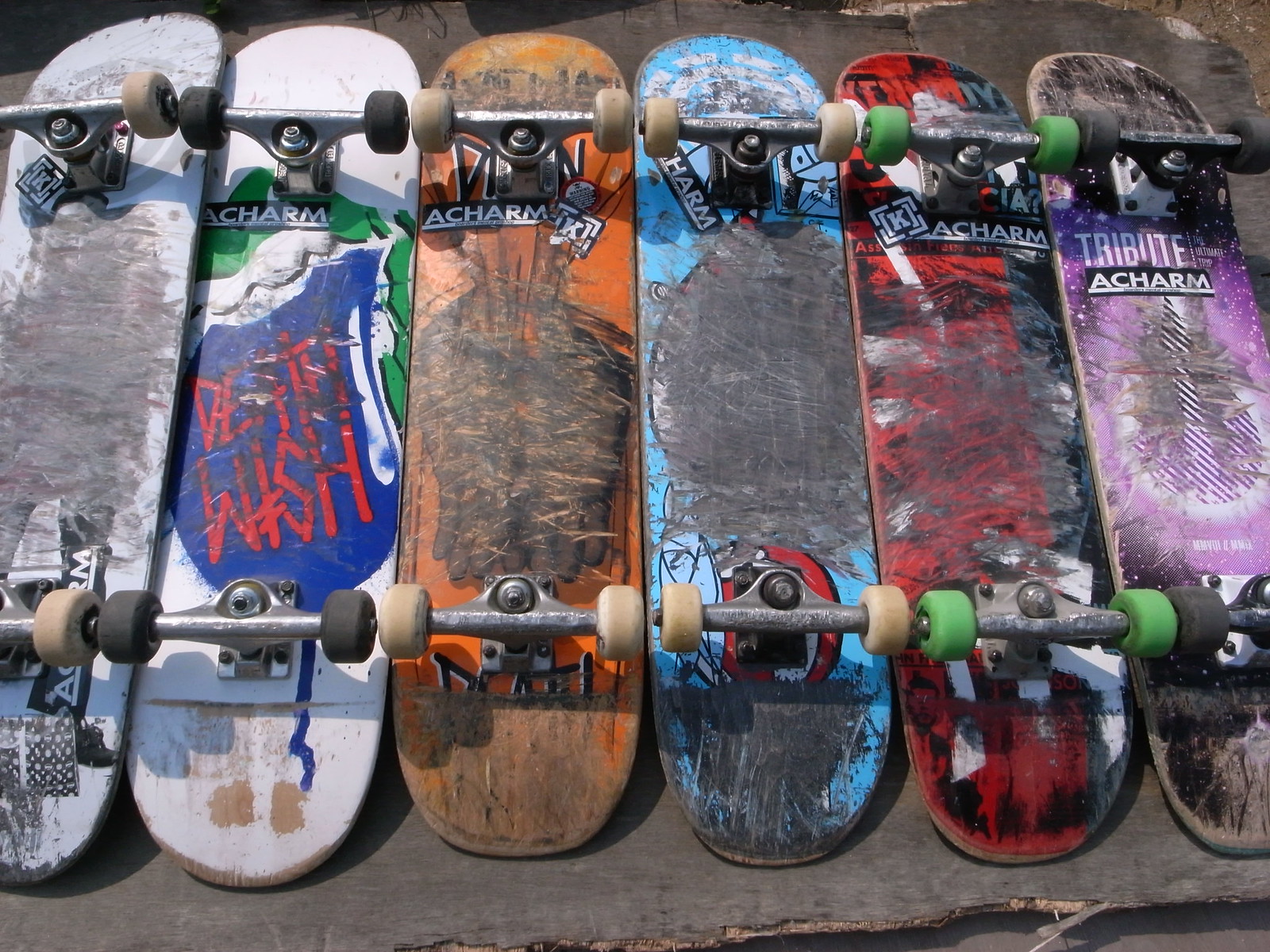This photograph captures the bottoms of six well-worn skateboards arranged closely together, with some overlapping. The skateboards, all lying on a dark, worn wooden surface, display a variety of heavily scraped and used designs, each telling a story of countless tricks and sessions.

Starting from the left, the first two skateboards are primarily white, with one having a notably scratched-out central design. The second board has a distinctive "Death Wish" text in red ink against a blue and white background, although much of it's obscured by wear. The third skateboard is bright orange, partly obscured by another board but featuring stickers that read "Akara." This "Akara" sticker, with white writing on a black background, is a recurring detail on almost all the skateboards.

The fourth skateboard is light sky blue, also with the main design mostly scratched off. The fifth skateboard combines red and black hues, and the sixth appears purple and black. Although the extensive wear and tear make it difficult to discern their original graphics, it’s evident these skateboards have been extensively used, showcasing the riders' dedication.

The wheels are as varied as the boards themselves; three skateboards sport cream-colored wheels, two have black wheels, and the red and black skateboard stands out with green wheels. This textured array of colors and layers against the background suggests a scene rich with skateboarding history and character.